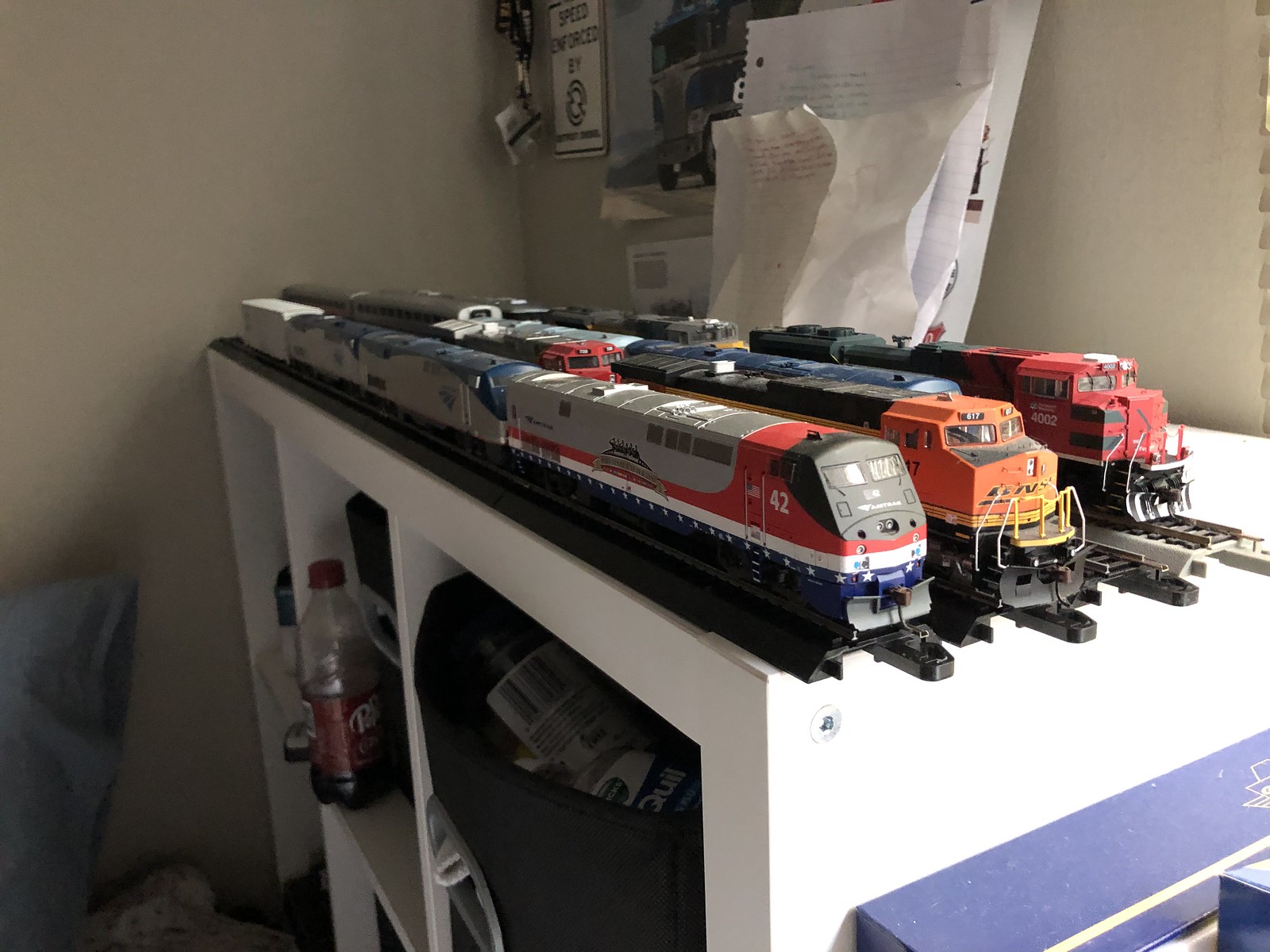The image features a white cabinet, resembling an Ikea Kallax unit, with multiple shelving compartments and model trains displayed on top. The trains are aligned diagonally from back left to front right, each on small plastic toy train track sections. The foremost train, decorated in red, white, and blue with an American flag and the number 42, is positioned closest to the camera. Directly behind it is an engine numbered 617 in orange, followed by a third engine numbered 4002, which is red and black. The trains each have four cars with varying colors, primarily gray, black, and mix-matched combinations.

The shelving unit underneath hosts a variety of items, including a small bottle of Dr. Pepper, a black bag containing medications like NyQuil, and assorted clutter. On the wall to the right of the cabinet, there are several pieces of lined notebook paper, pictures, a name tag key card, and a partially visible sign reading "speed enforced by". In the bottom left corner of the image, a beige-tan wall is visible, along with a blue pillow propped against it. The setting transitions from a brown wall on the left to a gray wall dominating the center and right of the background.